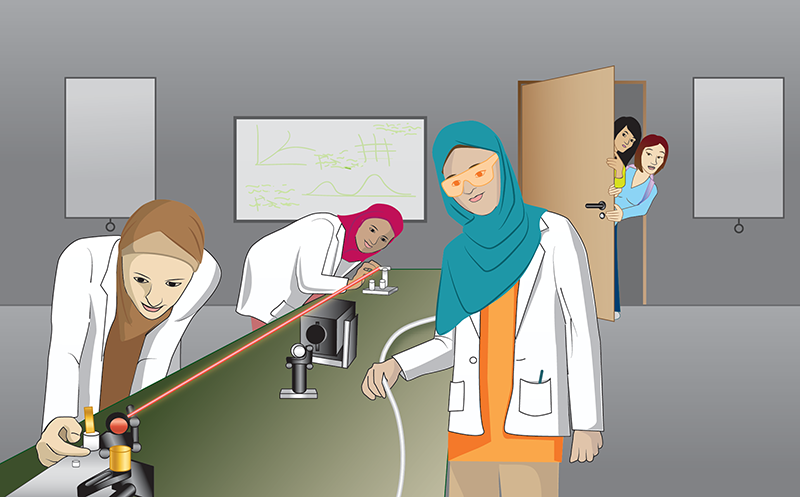The image is a horizontal rectangular drawing of a lab setting in a semi-realistic, semi-cartoon style. In the foreground, three women wearing hijabs and white lab coats are working at a large, green laboratory table filled with microscopes, samples, and lasers. The woman on the right is holding a white tube, possibly a laser, while the two women on the left are bent over their microscopes, closely examining samples. The lab features gray walls and a matching gray floor, with three window shades and a wooden brown door on the right side. The door is slightly ajar, revealing two people peeking in from the outside – a man and a woman, both only partially visible. The woman has black hair and wears a lime green shirt, while the man has reddish-brown hair, a blue shirt, and a purple-strap backpack. The background scene includes screens hanging on the wall, indicative of a typical scientific environment.